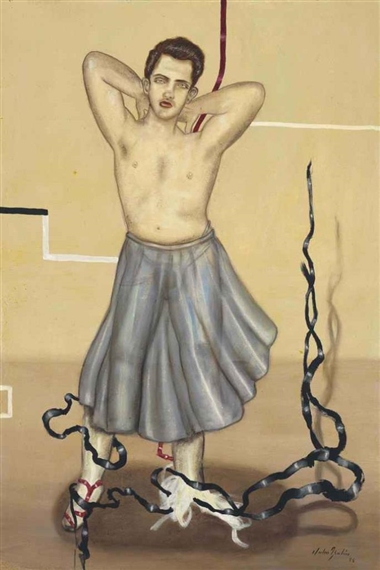This painting portrays a young man standing in an almost surrealistic and somewhat abstract setting, blending elements of both masculinity and femininity. The man, with short dark brown hair and a pale complexion, is primarily naked, but he wears a semi-transparent skirt that allows a veiled glimpse of his genitals, suggesting he's wearing a jockstrap underneath. His outfit is completed with red strappy sandals and red lipstick, enhancing his androgynous appearance.

The man stands with his arms raised, elbows pointing outward, and hands clasped behind his neck, as though he is admiring himself or lost in a moment of introspection. His posture suggests a sense of self-assurance and sensuality. Surrounding him are black and red ribbons that seem to float in midair, some trailing around his legs and rising up towards his arms, creating an enigmatic atmosphere that intertwines with the abstract and cubist background.

Overall, the painting captures a complex blend of sexual expression and self-reflection, inviting the viewer to contemplate the interplay of gender and identity.